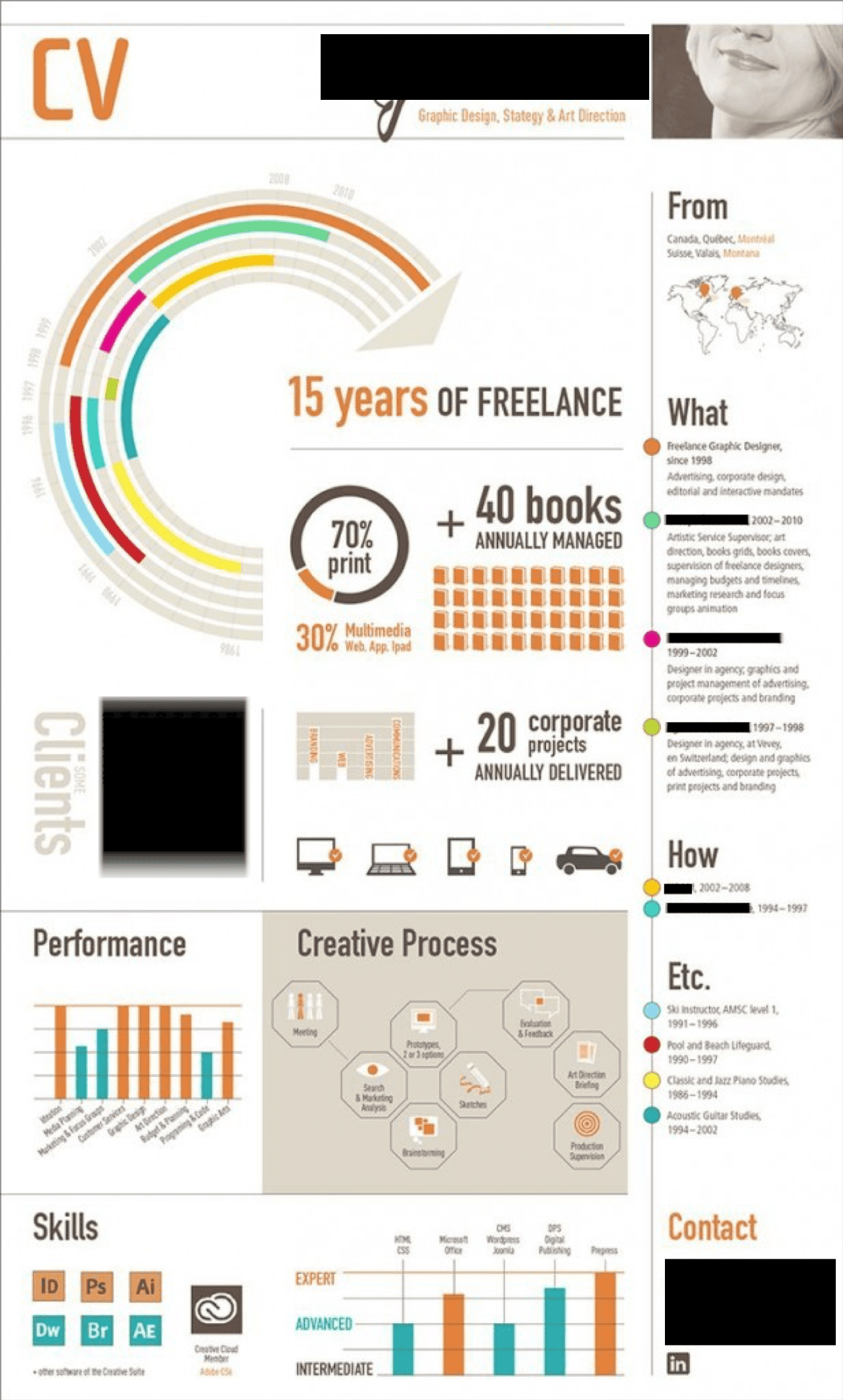The image is a detailed and visually rich poster that seems to be a comprehensive CV on a white background. Dominating the upper left-hand corner are the bold capital letters "CV" in orange. The poster highlights 15 years of freelance experience, with a pie chart depicting that 70% of the work is in print and 30% is in multimedia, alongside a statistic indicating the management of 40 books annually. The poster is a blend of text and various graphical elements, including a big wheel diagram, bar graphs, and numerous icons like a car, laptop, screen, and phone. It also discusses key competencies such as graphic design, strategy, and art direction, and provides an overview of the company's history, client types, and general creative process. There are two small maps indicating locations in Western Europe and a high point in North America, potentially Canada. Additionally, there's a blocked-off name section, and in the top right corner, a partial image of a smiling woman is visible, showing only her chin. The overall layout is sectioned with infographics, illustrations, and descriptive text, providing an insightful and engaging visual representation of the freelance work and achievements.